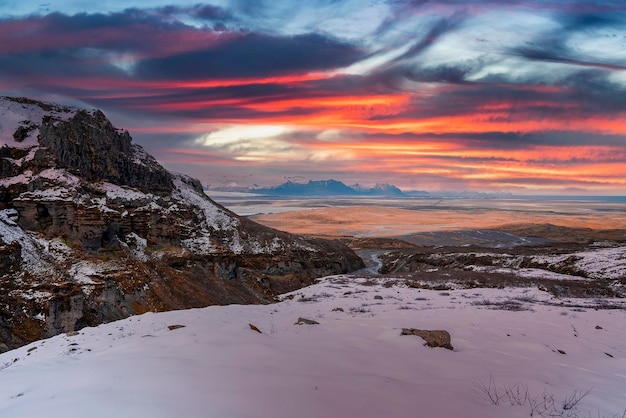The photograph captures a breathtaking sunset over a snowy, mountainous landscape, possibly in Alaska or Siberia. The sky is a vibrant tapestry of bright reds, yellows, pinks, and oranges, with clouds illuminated from below by the setting sun. Majestic mountains dominate the scene, their rocky, jagged cliffs cloaked in snow. In the foreground, a river winds through a flat, snow-covered area with exposed brown soil and interspersed rocks. The scene is framed by a cliff on the left side, while the distant horizon reveals a mountain range jutting up from a flat, prairie-like expanse. The valley below features barren, dry land intermingled with snow patches. Overall, the image beautifully combines the stark beauty of the snowy terrain with the dramatic colors of the sunset sky.